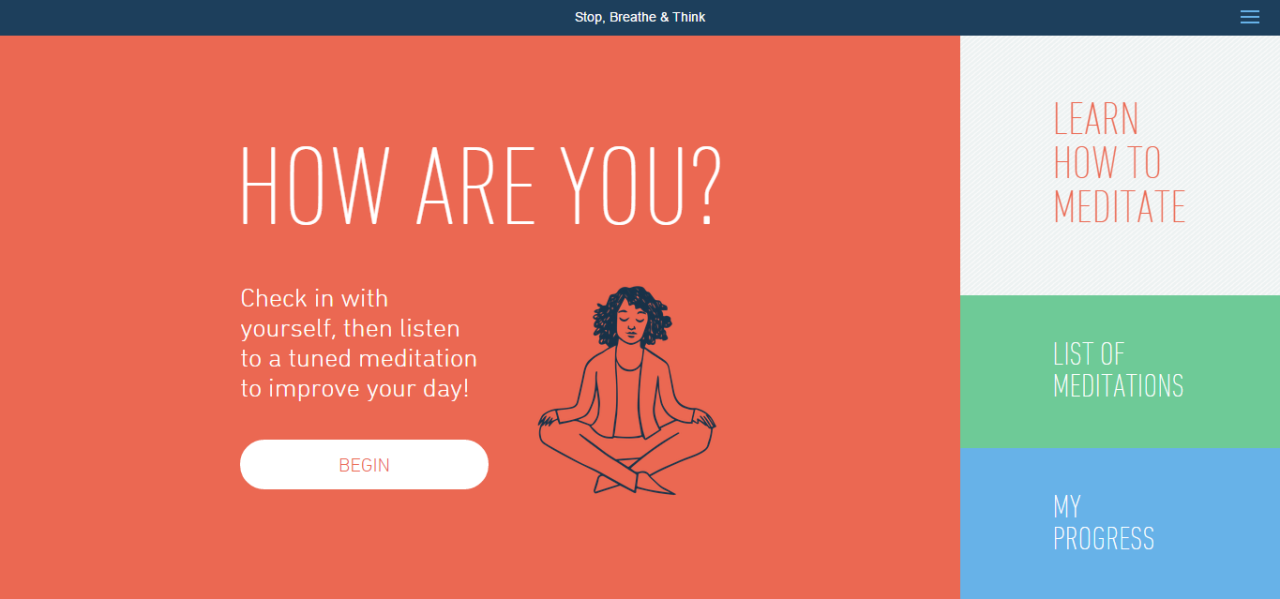The webpage features a calming, user-friendly interface designed to guide visitors through a mindfulness experience. At the top, a blue banner spans the width of the page, prominently displaying the phrase "Stop, Breathe, and Think" in the center, accompanied by a hamburger menu icon on the right.

Beneath the banner, the majority of the page is filled with an orange section that immediately asks, "How are you?" On this orange background, there's a simple, stylized illustration of a woman sitting in a lotus position, symbolizing meditation and tranquility. The text encourages users to "Check in with yourself, then listen to a tuned meditation to improve your day!" To facilitate this process, a prominent white "Begin" button is situated below the text, inviting users to start their mindfulness journey.

To the right of this central content, three vertically aligned boxes offer additional options. The top box is white, featuring the text "Learn How to Meditate." The middle box, colored green, provides a "List of Meditations." The bottom box is blue and titled "My Progress," allowing users to track their meditation journey.

Overall, the webpage combines soothing colors, intuitive design, and clear calls to action to support users in achieving mindfulness and improving their well-being.